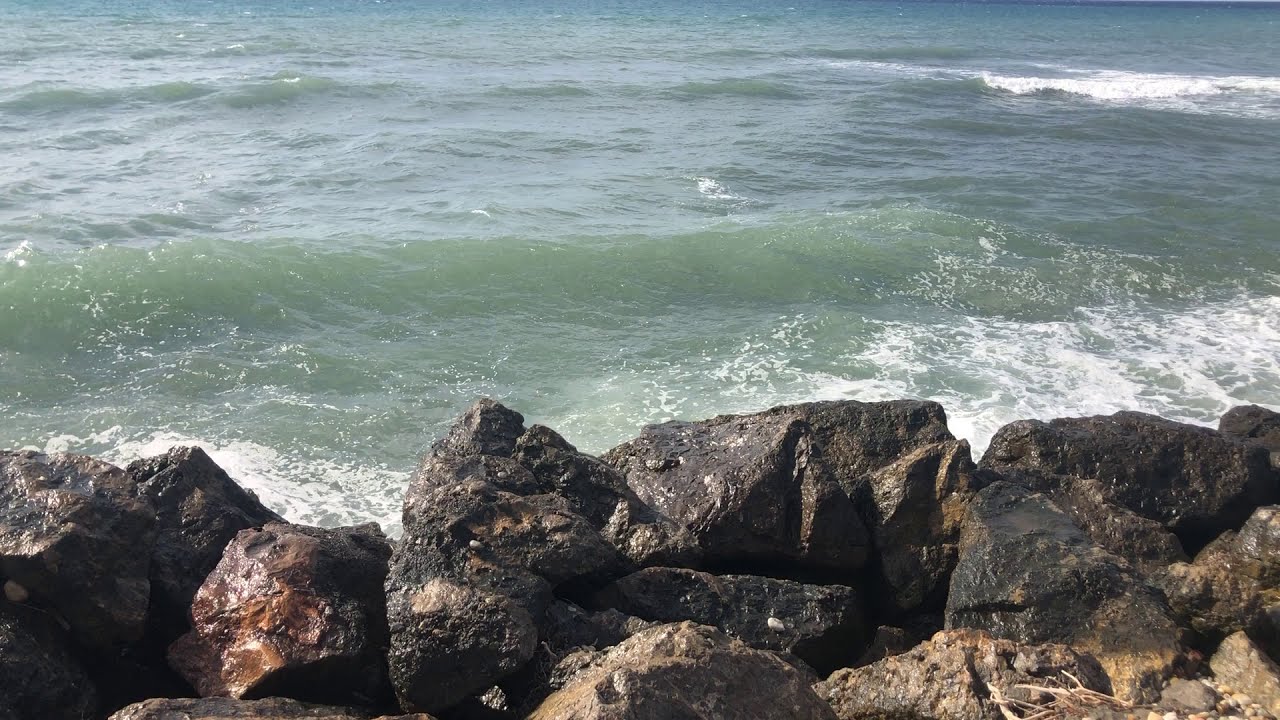The photograph captures a dramatic oceanic shoreline scene during daytime. At the forefront of the image, there is a tightly piled collection of approximately a dozen giant boulders, varying in color from dark grays to dark reds, many of which are wet and glistening while some remain dry towards the bottom right corner. These jagged, rugged rocks form a natural cliff that offers a vantage point for gazing out over the seascape. The ocean stretches out behind the rocks, with waves crashing vigorously against them. Two distinct waves are approaching, the closest one showcasing a captivating seafoam green tint with hints of clear jade that transforms into frothy white upon impact with the boulders. Another wave, curling over, adds to the dynamic motion in the upper right corner of the image. The water, a blend of murky bluey-green closer to shore and transitioning to a deeper, more pronounced blue at the horizon, conveys the forceful, turbulent nature of the sea. Small patches of possibly lighter-colored seaweed can be seen amongst the rocks, adding additional texture and depth to the shoreline. At the top of the photograph, a thin strip of deep blue sky completes the color palette, emphasizing the ocean's vastness and the rugged beauty of the coastal scene.